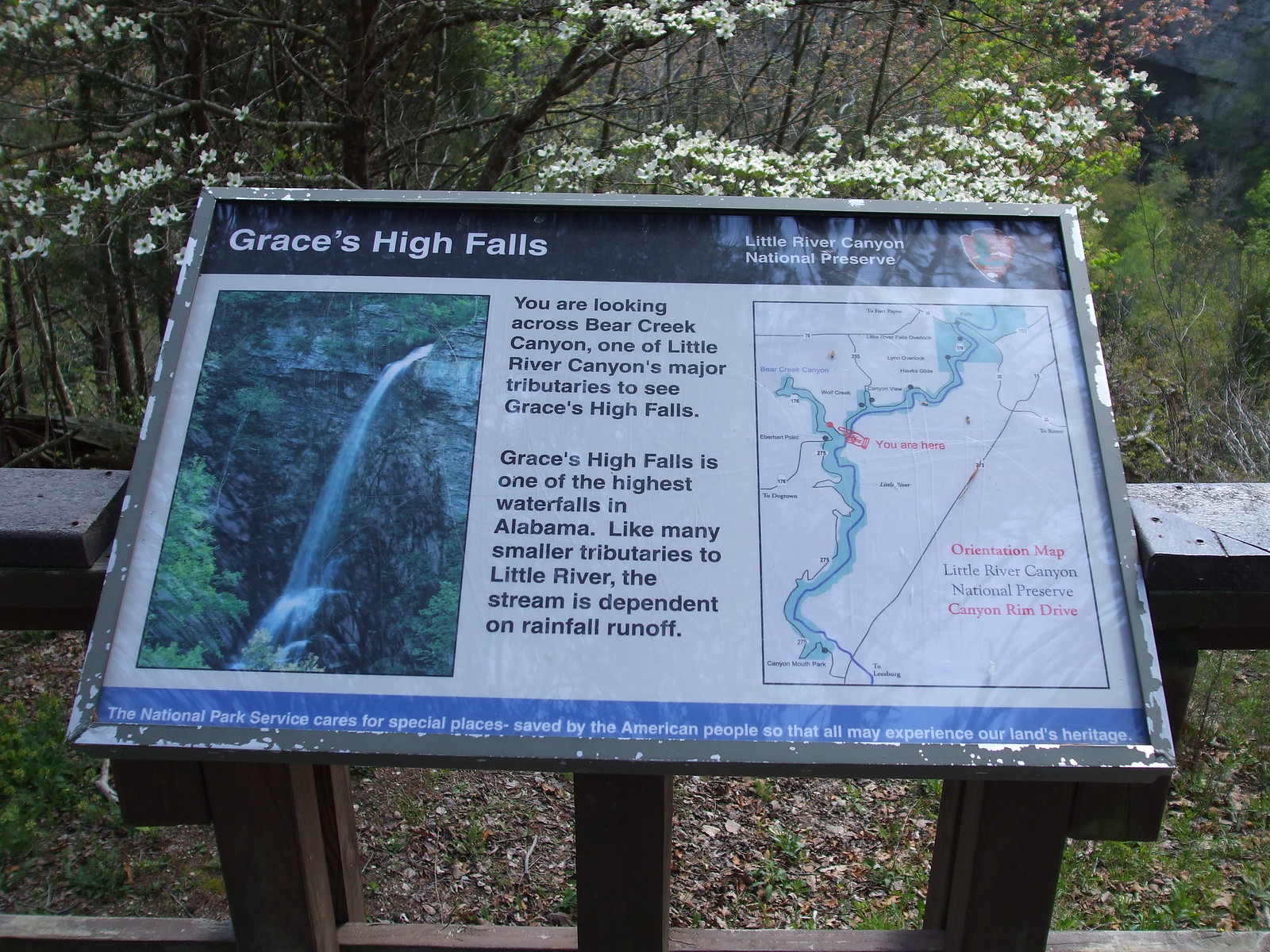This image showcases an informational plaque set against a wooden railed fence in a forested area. The plaque is marked by a wide black strip across the top, reading "Grace's High Falls" in the upper left corner and "Little River Canyon National Preserve" in the upper right corner, alongside a National Parks logo featuring red and green shield colors. Below this, the left side of the plaque features a large, vibrant photograph of Grace's High Falls—a majestic waterfall tumbling over a rocky precipice amidst surrounding trees. Adjacent to the photograph, black text provides details: "You are looking across Bear Creek Canyon, one of Little River Canyon's major tributaries, to see Grace's High Falls. Grace's High Falls is one of the highest waterfalls in Alabama. Like many smaller tributaries to Little River, the stream is dependent on rainfall runoff." On the right side of the plaque, there is an orientation map of Little River Canyon National Preserve's Canyon Rim Drive. The plaque is elegantly enclosed within a wooden case, adding to its rustic charm. The area around the plaque is rich with natural elements—dirt, leaves, grass, wild white flowers, and a backdrop of trees, evoking the serene beauty of the national reserve.